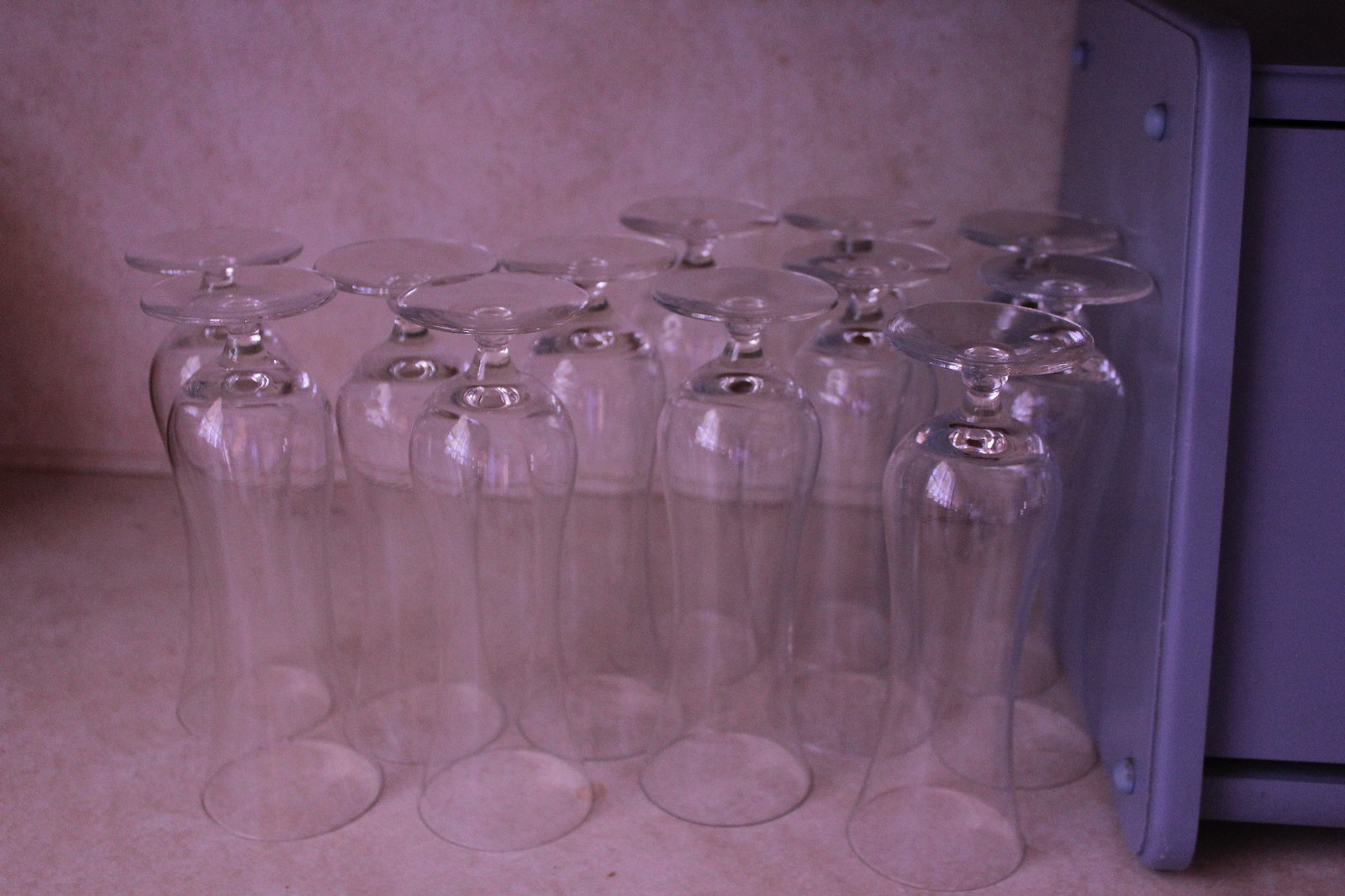The photograph features 12 clear, long-stemmed glasses with a wide bottom, arranged upside down on a countertop, as if drying. The glasses are set on a surface that resembles a pinkish or rosy marble-laminate pattern, extending to the backsplash with the same design, evoking a 1950s or 60s aesthetic. Positioned somewhat haphazardly yet in discernible clusters, the glasses are organized into three rows: three in the back row, five in the middle, and four in the front row. To the right of the glasses, a bluish-purple rectangular bread box with two knobs on one side is partially visible, adding a splash of color to the setup. The bread box and its detailing suggest a simple, functional design.